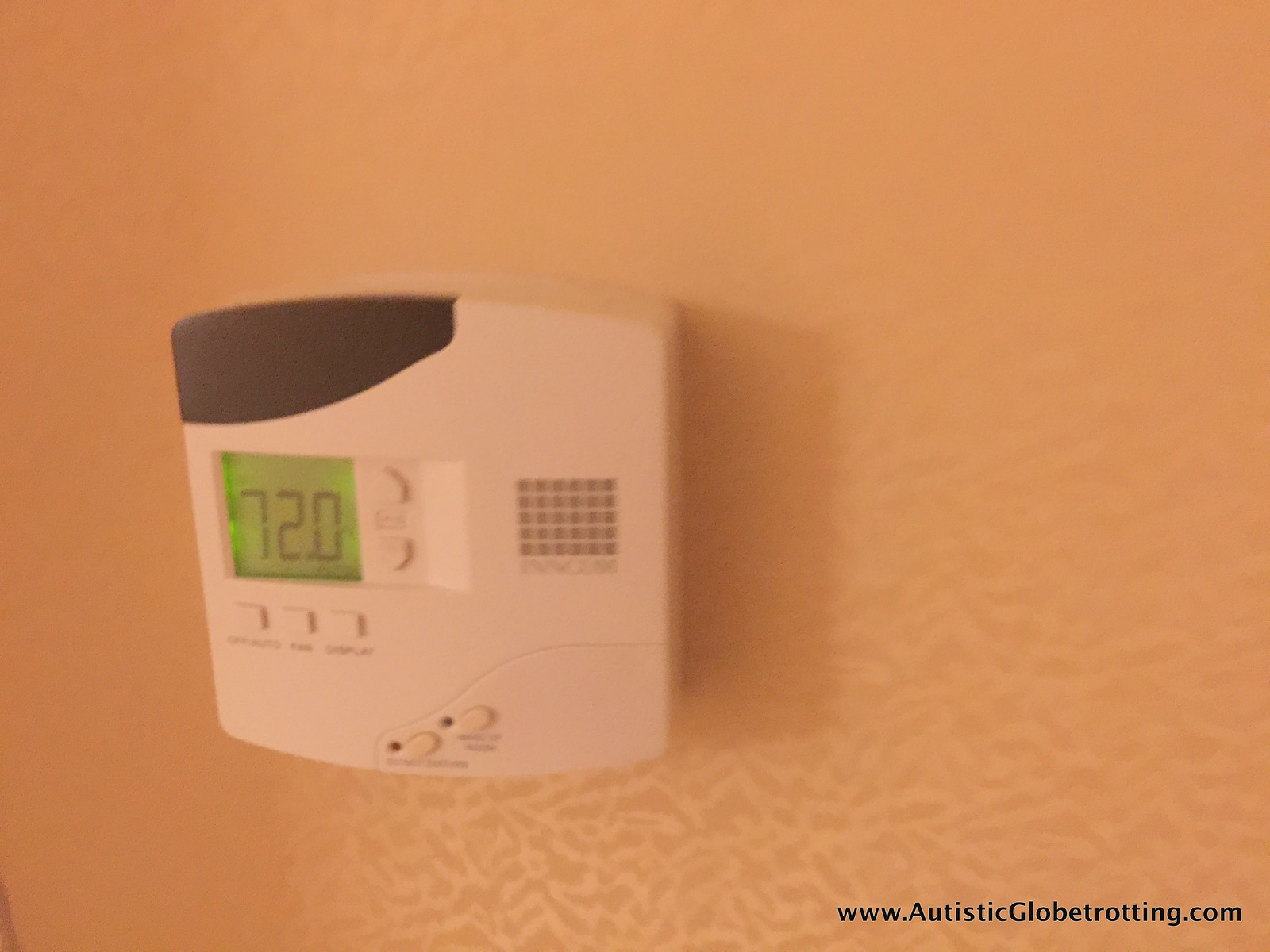The image features a predominantly orange background that exhibits a subtle, intricate pattern at the bottom and along the right edge, consisting of lighter orange, squiggly lines over a darker orange backdrop. Centrally, there is a temperature control device in a light pinkish-orange hue, adorned with various elements. On the upper left of the device, a brown shape is present, and a green display window prominently shows the number "720." Adjacent to this window are two barely noticeable buttons in the same color as the background, distinguishable only by their shadows.

Below the green window, three additional buttons are arranged horizontally, featuring unreadable text beneath them. To the right of these buttons, a red dot accompanied by a wave pattern and a black dot labeled with the number "2" can be seen, followed by more text that is too small to decipher. Further down, a rectangular area composed of small brown squares is present, with more illegible text beneath it. In the lower right-hand corner of the image, the text "www.autisticglobetrotting.com" is clearly displayed.